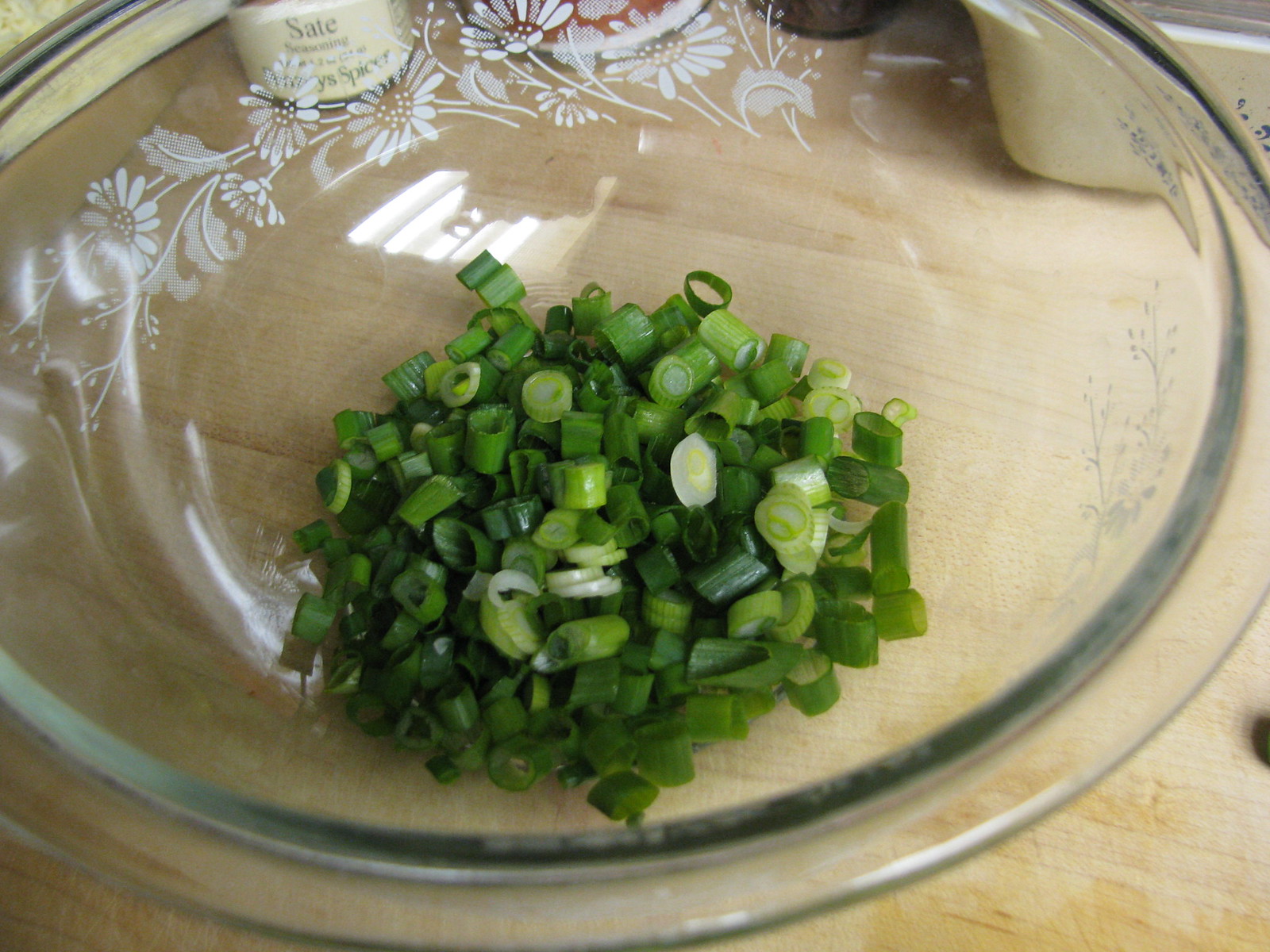The image showcases a transparent glass plate adorned with intricate white floral patterns, featuring petals, stems, and swirling flourishes. Captured from a top-down perspective, the plate rests on a yellowish-brown wooden work surface, enhancing the clarity of the glass and the delicacy of the floral design. Centered on the plate, a meticulous pile of finely diced green onions, with their vibrant green and white hues, stands out starkly, infusing the scene with a burst of color. In the background, a glass baking dish, a white ceramic casserole dish, and a small jar labeled "satay seasoning spices" are visible, adding depth and context to the rustic kitchen setting.